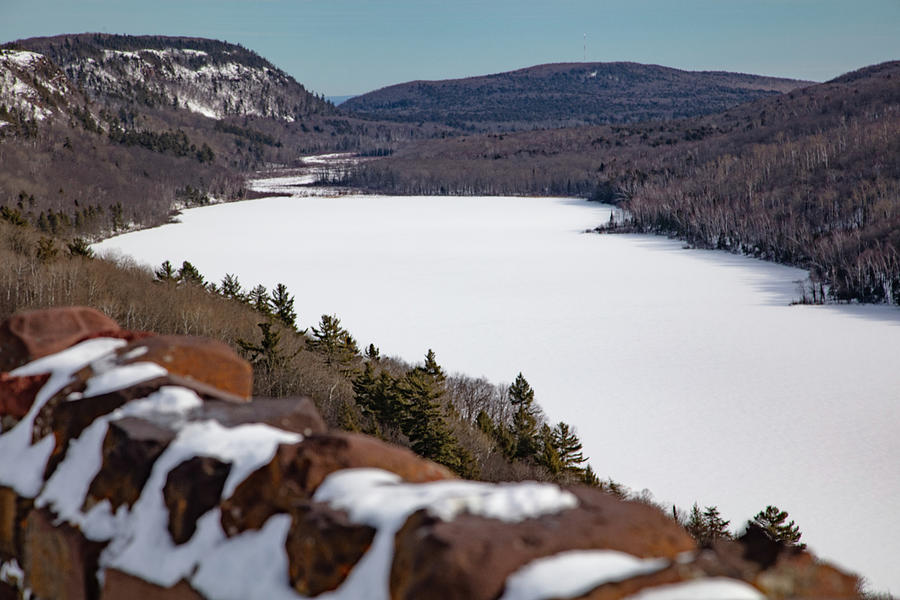The photograph captures a breathtaking winter scene from a high vantage point, likely taken from a roadway above. In the foreground, a rock wall made of dark gray and terracotta stones dusted with snow runs along the lower left side of the image. Below the wall, the focus shifts to a wide, winding river that meanders from just left of center to the lower right-hand corner, completely frozen over and blanketed in snow. On both sides of the river, the landscape is dotted with a mix of barren trees and evergreen pines, which retain their green needles. The setting extends into a serene valley flanked by snow-capped mountains, mostly adorned with pine trees. The clear blue sky above suggests a bright, sunny winter day, casting light on patches of melted snow on the trees and enhancing the natural beauty of this northern, cold climate scene.